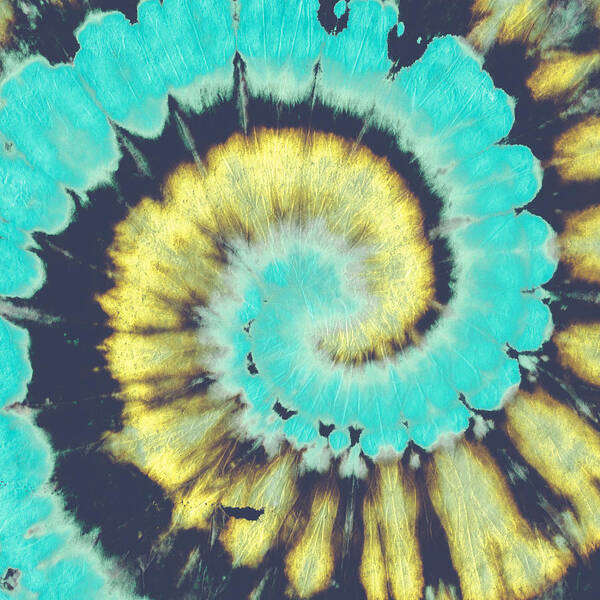This vibrant and artistic image features an intricate, colorful pattern reminiscent of a tie-dye t-shirt or the mesmerizing view through a kaleidoscope. At the center, a swirling mix of turquoise, blue, and green colors spiral outward, creating a dynamic focal point. Surrounding this core, bright yellow hues radiate towards the edges, providing a striking contrast. Darker bands of navy blue or black intricately split and accentuate the lighter colors, further enhancing the spiral effect. The composition resembles a close-up of a flower, capturing an essence that is both natural and abstract. The pattern's vivid and harmonious interplay of colors—ranging from light blue to dark blue, yellow, turquoise, and green—captures the eye with its burst of brightness and artistic elegance, making it an image worthy of display in a gallery or an affluent living room. Notably, the image is free of text, emphasizing its pure visual impact.